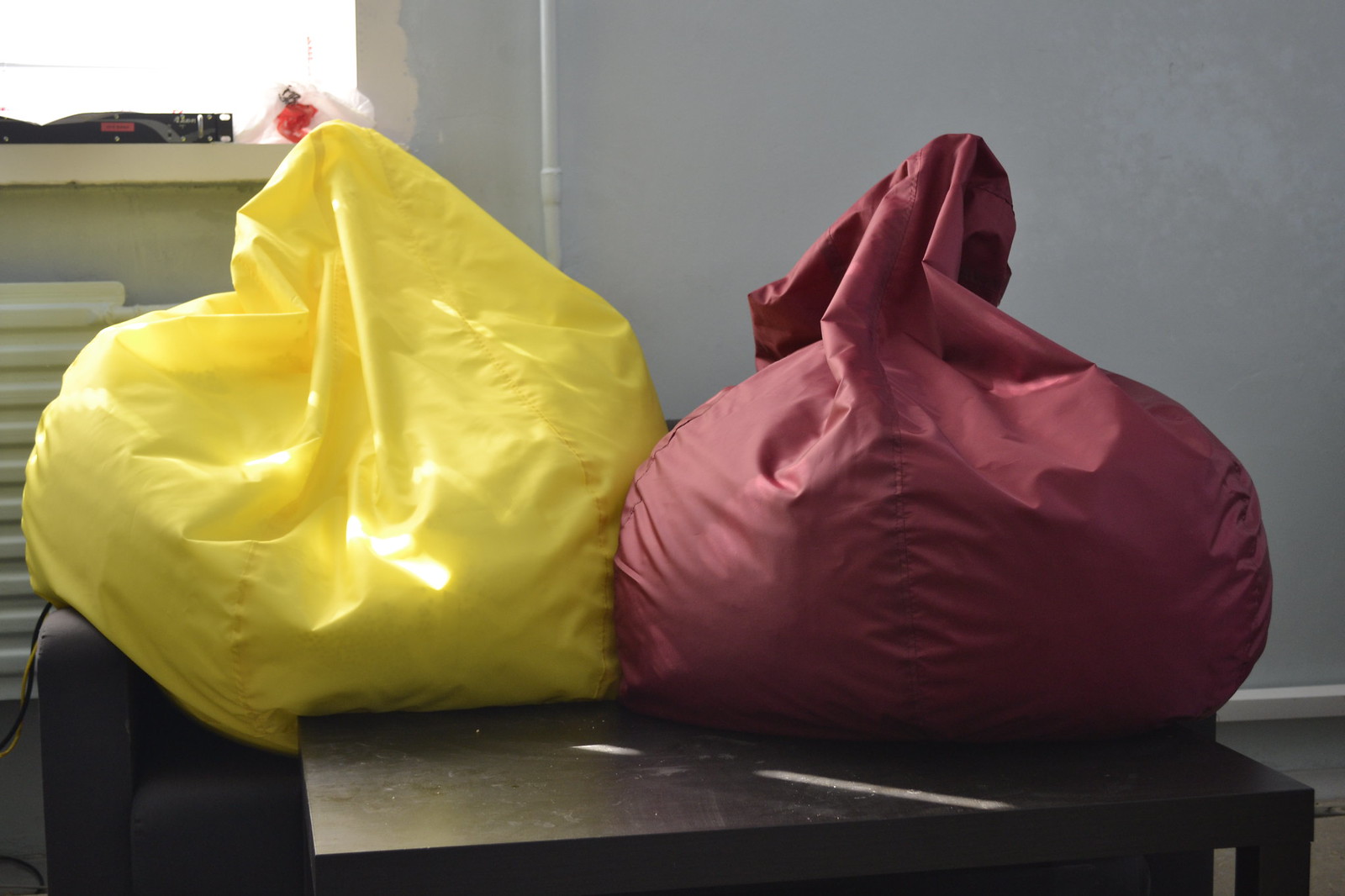The image depicts a relatively cluttered, makeshift lounge area that looks like it might be in a college dorm room or casual living space. Central to the scene is a black Ikea Lack coffee table, visibly dusty and smudged. Behind this table is a black futon or sofa, partially obscured by two beanbag chairs—a burgundy one and a yellow one—haphazardly bunched up on the couch. The surrounding environment features a bluish-gray wall with some unfinished white paint marks around a window ledge, partially visible in the upper left of the photo. Additional details include a white pipe extending upward along the left-middle part of the wall, some wires trailing from the bottom left of the couch, a white baseboard trim along the bottom of the wall, and a grayish carpeted floor. The overall scene appears somewhat disorganized, with hints of neglect and everyday clutter.